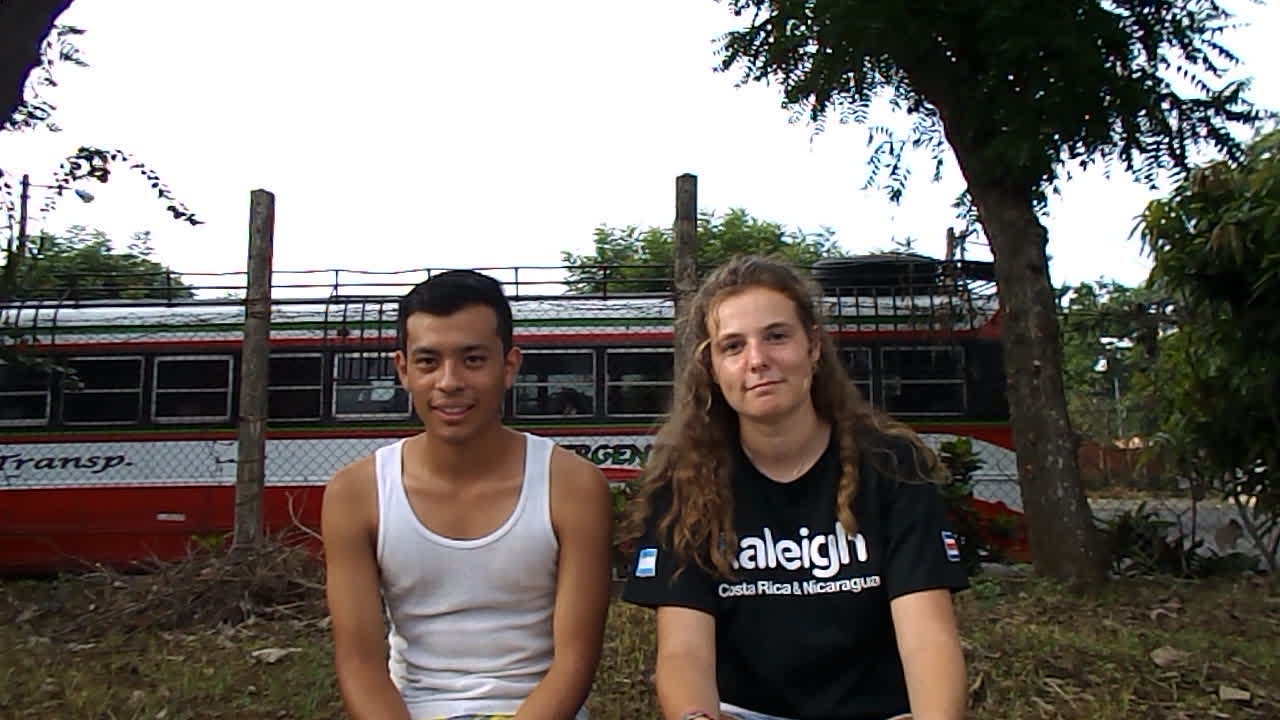In this photograph, two young people, possibly in their late teens or early twenties, are sitting next to each other and smiling at the camera. The young man on the left has dark skin and short, cropped dark hair, suggesting he could be of Latino or Indian descent. He is wearing a white tank top. The young woman on the right is Caucasian with long, curly brown hair. She is wearing a black t-shirt with the words "Raleigh" prominently displayed, followed by "Costa Rica" and "Nicaragua" in smaller lettering. Her shirt also features the flags of these two countries on the sleeves.

They appear to be sitting on a bench or a low structure in an open, grassy area that has patches of dirt and leaves scattered around. Behind them, there is a makeshift fence and some posts. Further in the background, a white bus with red stripes and black windows is visible. The bus has the word "Trans-P" written on its side, along with green writing and green racks on its silvery rooftop. Trees and shrubs frame the background, with the bright sky peeking through the foliage. This posed photograph captures a clear, sunny day with a relaxed, tourist-like atmosphere.